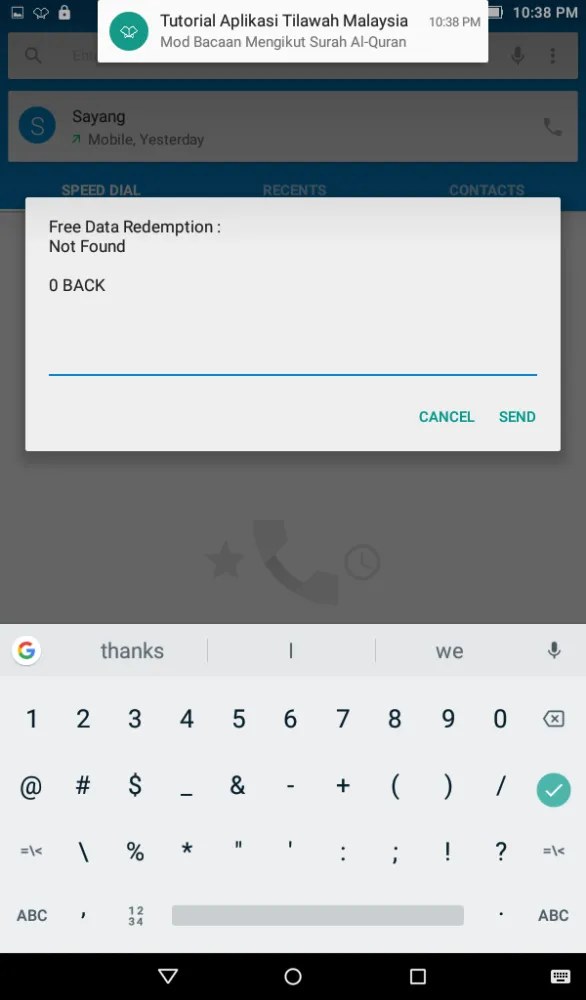The image is a detailed screenshot from a mobile phone tutorial viewed at 10:38 p.m., presumably in Malaysia, as indicated by the text "Apalikasi, Tawala, Malaysia" at the top of the screen. The phone's interface displays the time as well, confirming the late hour. In the upper part of the screen, an icon with what appears to be wings inside a green circle is visible. The background of the screenshot is grayed out, suggesting that an overlay or pop-up is currently active.

The overlay lists various options, including "Sayang Mobile yesterday," "Speed Dial," "Recents," and "Contacts." At the topmost portion, there is a tab that indicates the presence of additional content. The active pop-up prominently features the message "free data resumption" followed by a semicolon with no further text. Below this, the words "not found" are displayed, followed by a thin blue bar spanning the width of the pop-up and a space labeled "zero back." At the bottom of the pop-up are two green buttons labeled "cancel" and "send," positioned to the left and right, respectively.

Further down the screen, the phone's keyboard is visible, currently displaying numbers and symbols instead of the typical alphabet. The keys show numerals from 1 to 0 and special characters such as @, #, $, _, &, etc. On the far right of the second row of the keyboard, a green circle with a white check mark inside is prominently displayed. The keyboard also features a space bar, capitalization options, and a basic navigation bar at the very bottom with the standard triangle, circle, and square icons, as well as a keyboard icon on the far right. The navigation bar is solid black, providing a stark contrast to the other elements on the screen.